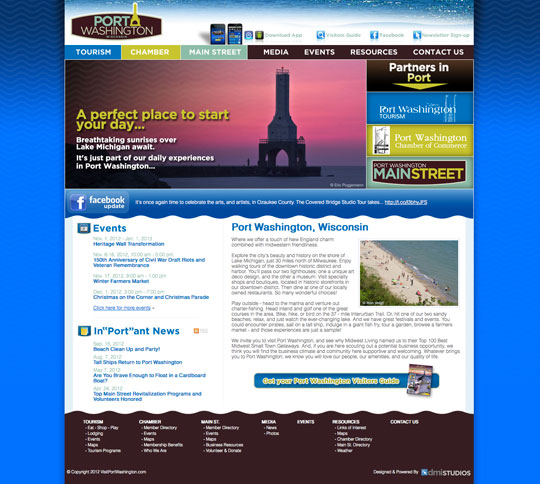The image showcases the website of Port Washington, prominently displaying the title "Port Washington" at the top. The words "Port" and "Washington" are both capitalized, with "Port" bolded for emphasis. Adjacent to the title, there appears to be an insignia resembling a tower. Below the title, a navigation bar lists categories: Tourism, Chamber, Main Street, Media, Events, Resources, and Contact Us.

The background of the website is a calming blue, with bordered sections on both the right and left sides. Under the navigation bar, an image of what appears to be a lighthouse is accompanied by the gold-colored text, "A perfect place to start your day..." followed by additional informational text. 

Further down, a wavy blue banner with a Facebook update contains white text at its center. Below this banner, the section titled "Events" is bordered by five lines of blue text, which are unreadable due to their small size. The "Important News" section follows, marked by an icon to its left and four lines of blue content that are similarly hard to read.

In the middle of the page, the words "Port Washington" reappear, introducing an article that spans about four paragraphs. Next to the article is a media image depicting a beach, with additional, albeit unreadable, information located beneath it.